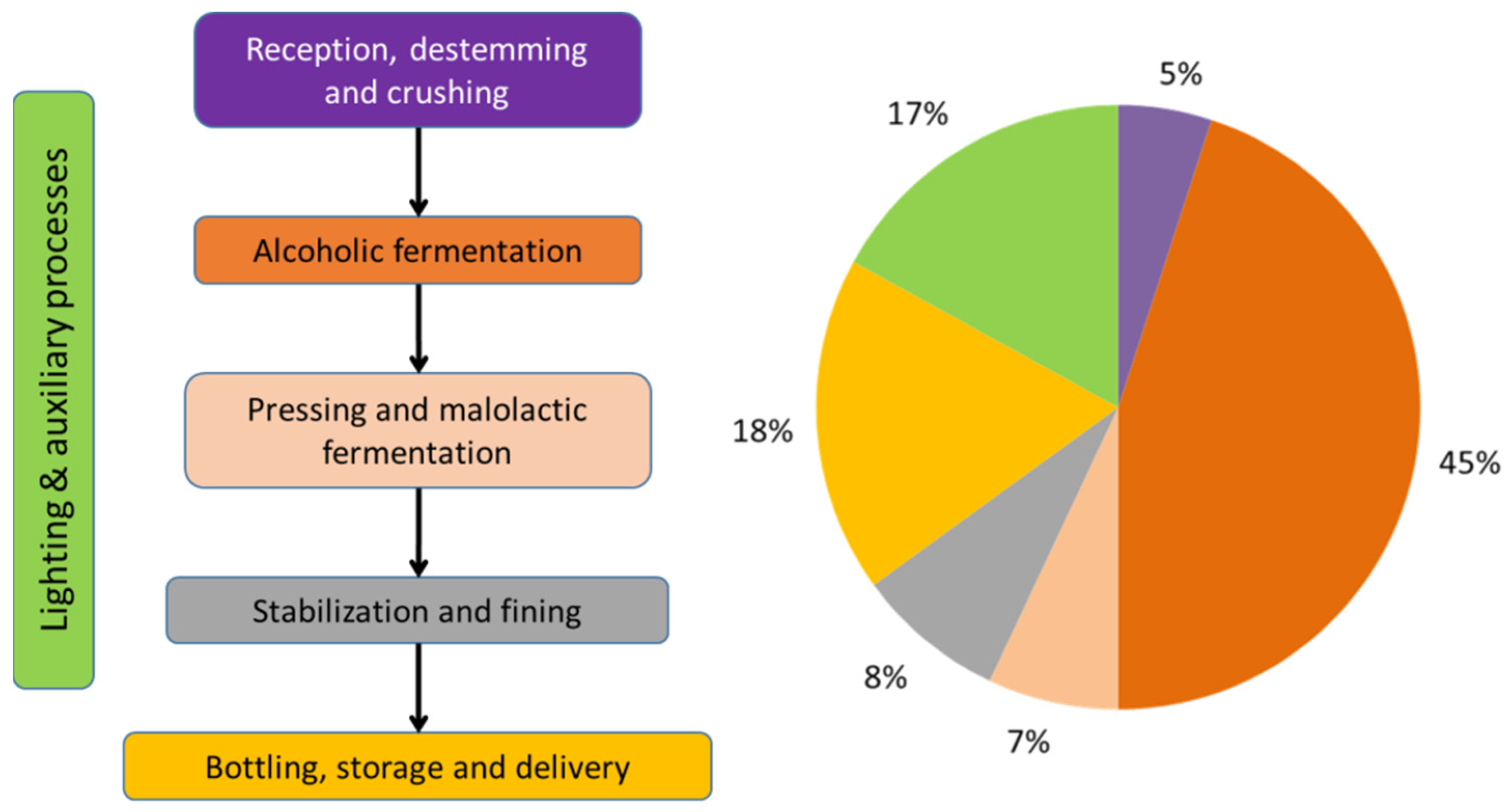Here is the cleaned-up and descriptive caption for the image:

---

The image displays a detailed graph chart, with a prominently featured pie chart located on the right side. The pie chart is segmented into various colors representing different processes and their corresponding percentages: 5% purple, 45% orange, 7% tan, 8% gray, 18% yellow, and 17% green.

Each color on the pie chart is associated with specific stages in the production process:
- 5% Purple: Reception
- 45% Orange: Alcoholic Fermentation
- 7% Tan: Pressing and Malolactic Fermentation
- 8% Gray: Stabilization and Fining 
- 18% Yellow: Bottling, Storage, and Delivery
- 17% Green: Lighting and Auxiliary Processes

On the left side of the chart, the green category of Lighting and Auxiliary Processes is highlighted separately.

The graphic chart succinctly outlines the different stages of the production process, with all its elements depicted in an upright and organized manner.

---